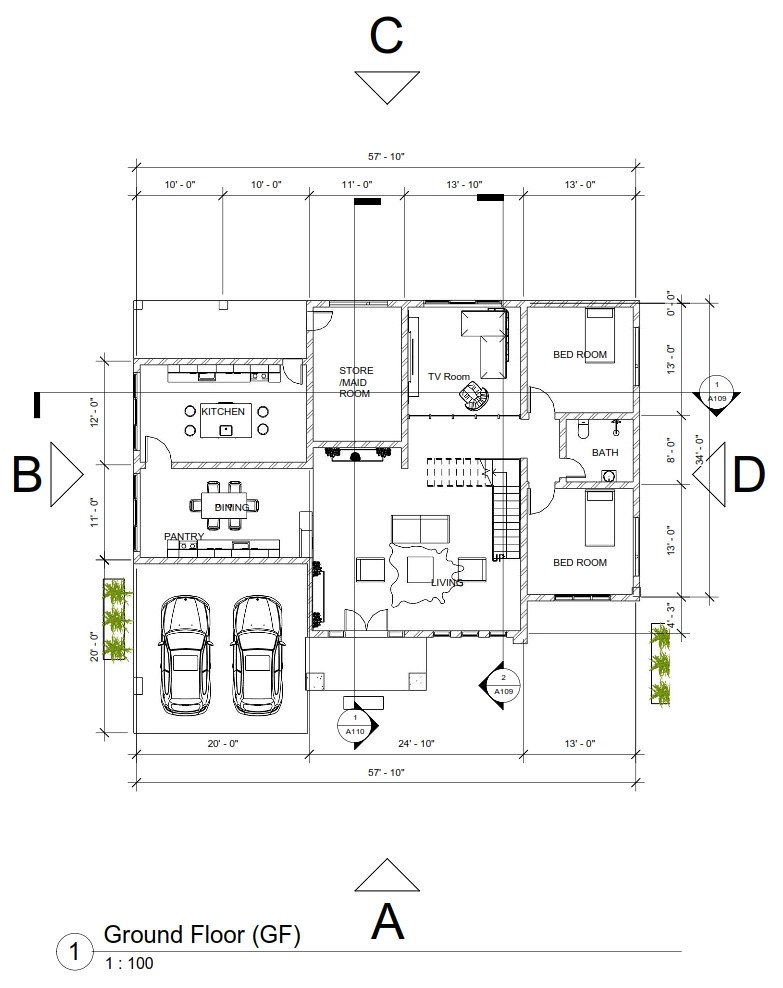This detailed architectural blueprint showcases the ground floor layout of a house. On the bottom left corner, a circled number "1" in black indicates the starting point, from which a straight black or dark blue line extends across to the right. Above this line, on the left side, the label "ground floor" is prominent in dark lettering. Centrally along this line, a large "A" with an upward-pointing arrow marks a significant focal point.

The blueprint illustrates a comprehensive floor plan featuring multiple rooms, labeled for clarity. Towards the top, the notation "bedroom" indicates the sleeping quarters. Adjacent, the living room, bathroom, additional bedroom, TV room, storeroom, and kitchen are meticulously drawn, all annotated and presented in precise blue or black ink on a white background.

Significant directional arrows are present throughout the blueprint: at the top, a "C" with a downward-pointing arrow; on the left, a "B" with an arrow pointing to the right; and on the right side, a "D" with a leftward arrow. The layout includes detailed measurements, numerical annotations, and schematic furniture arrangements to visualize the room setups effectively.

The image also depicts two cars positioned within the garage space, providing a realistic perspective of the area. Additionally, shrubbery is illustrated outside the garage door on the left, adding a touch of natural landscaping to convey the exterior aspect of the house design.